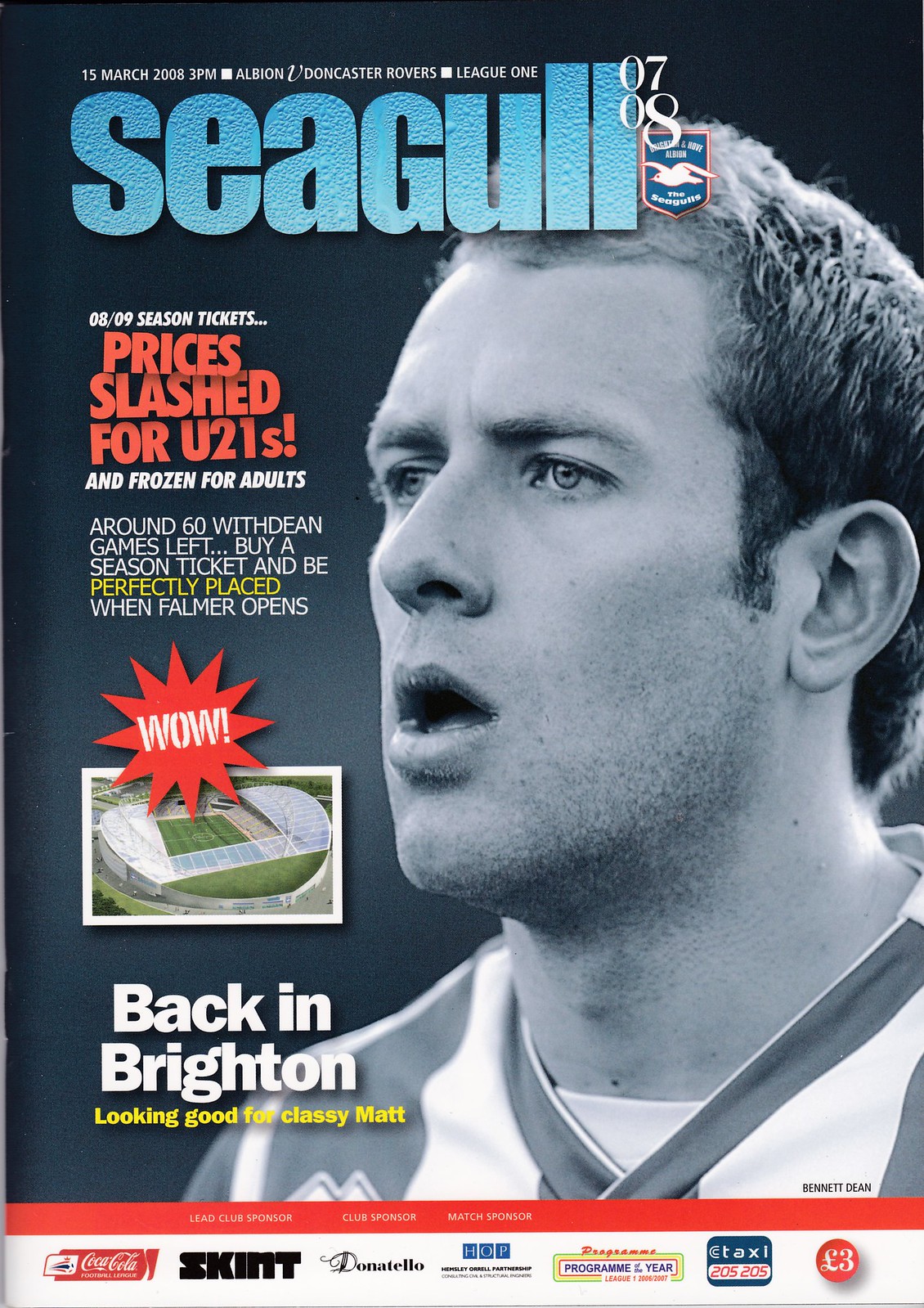This is the front cover of a sports program for a game between Albion and Doncaster Rovers in League One, held on 15 March 2008 at 3 PM. At the top, in large blue text, it says "Seagull 0708," with the numbers overlapping the last 'L'. The background features a close-up black-and-white photograph of a soccer player's face, wearing a V-neck jersey. The player has an open mouth, forming an 'O', and eyes staring off to the side, giving him a shocked or surprised expression. To the left of his face, text highlights season ticket offers: "08/09 season tickets prices slashed for U21s and frozen for adults." There is additional text promoting that prices are frozen and season tickets could place fans in prime position when the new Falmer stadium opens. Also, there is a small image of a modern stadium with a star that says "WOW" over it. At the bottom left, a headline reads "Back in Brighton, looking good for Classymet." A row of sponsorship logos runs along the bottom edge of the cover.